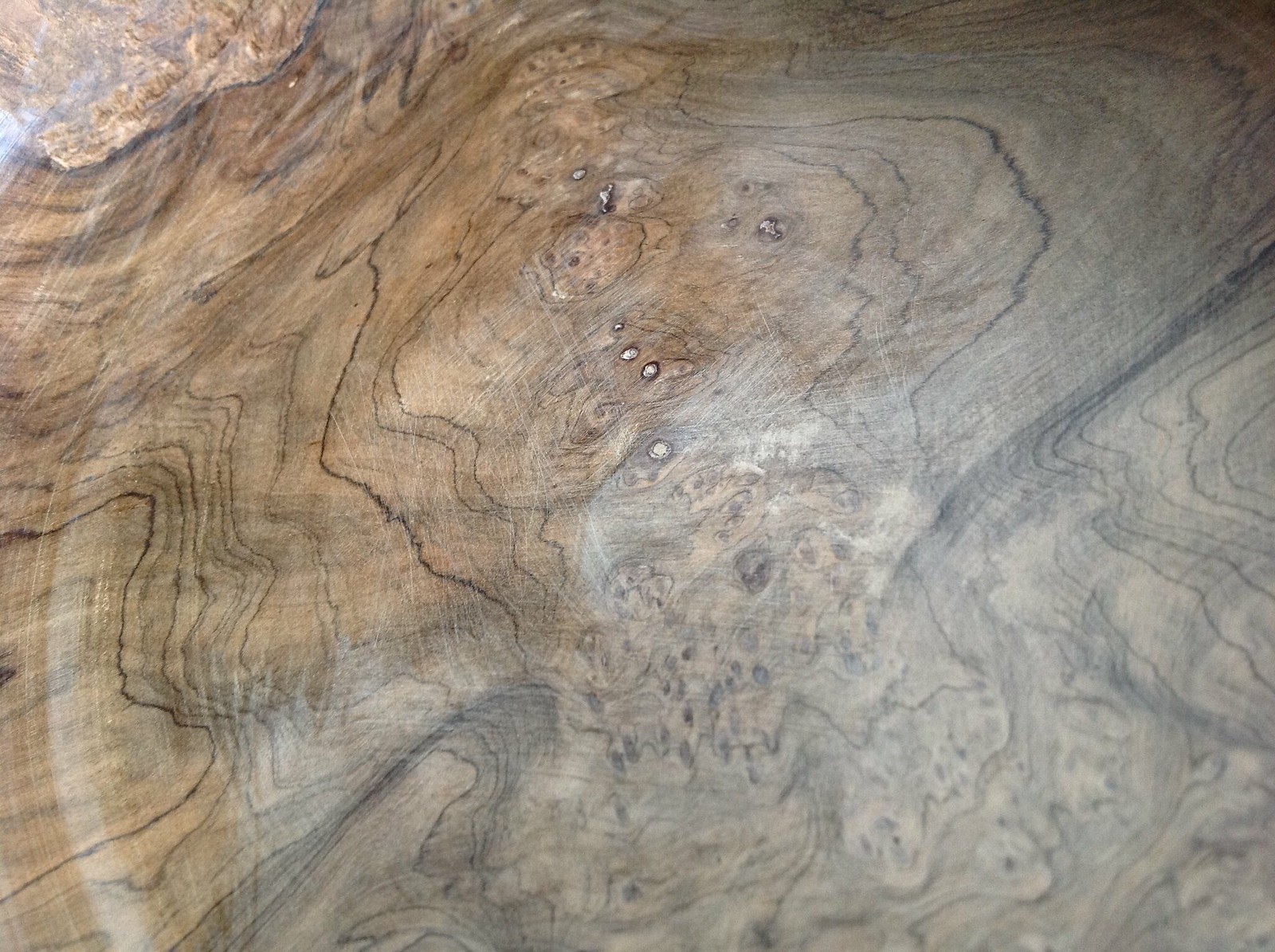This is a close-up photograph of a sliced section of polished wood, possibly from a tree trunk that has been made into a table. The intricate woodgrain patterns are visible, showcasing an array of dark lines and irregular rings that traverse the surface, resembling a topographic map or the look of dried-up riverbeds seen in aerial photos. The colors range predominantly from light brown to light gray, with patches of dark brown and white. In the center of the image, there are at least four dark-edged circular burn marks aligned in a row, with a few more scattered slightly to the left and right. The right side of the picture appears gray and washed out, while the left side retains its brown hue, though it seems to be fading. The non-uniform rings suggest the tree experienced considerable trauma during its growth. Additionally, the surface features several small white specks and a notable knot near the center, further adding to the detailed texture of the wood.